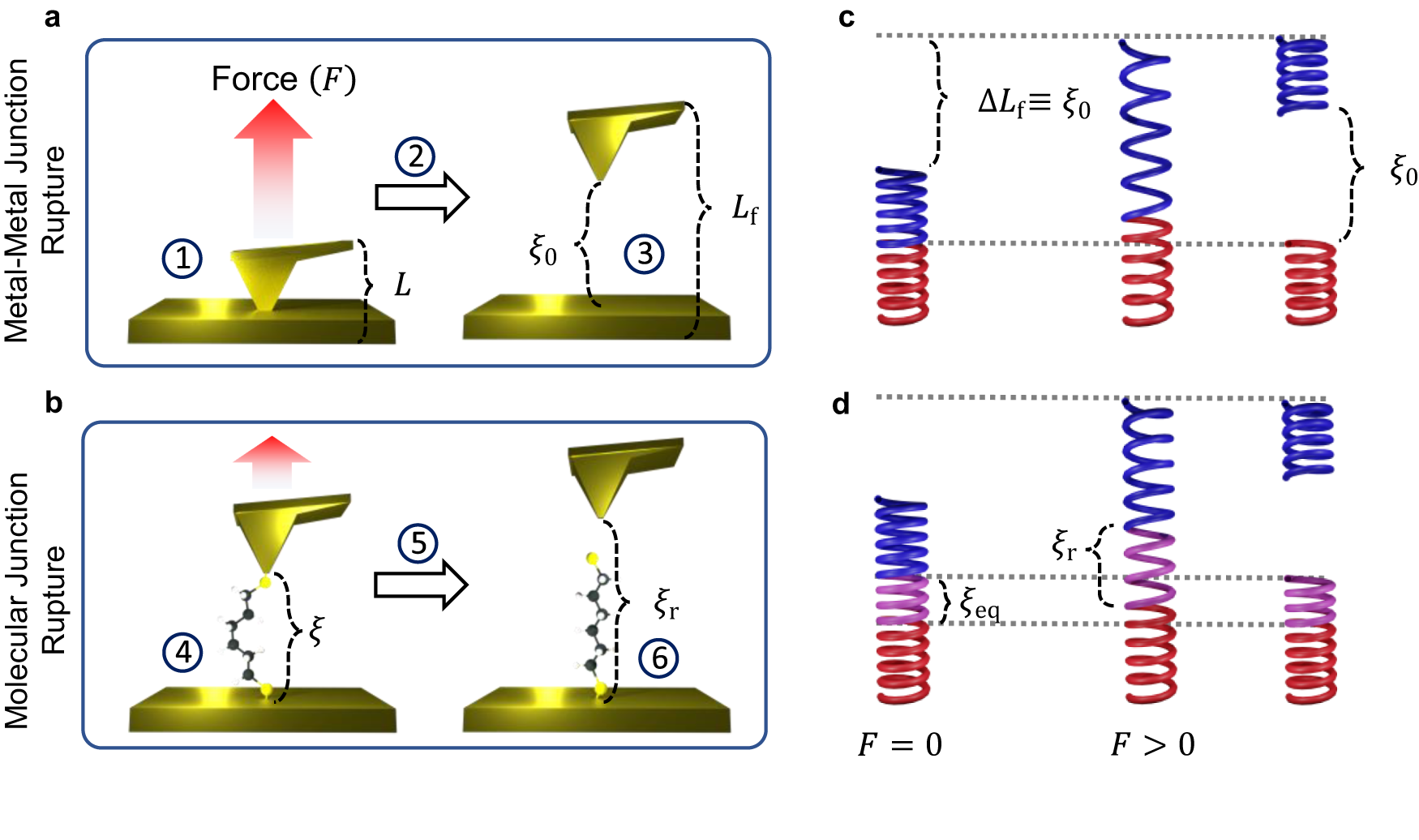This image is a detailed scientific illustration, likely from a physics textbook, featuring vivid colors and various mechanical and electrical components. On the left side, there are two gold rectangular diagrams labeled "A" and "B." Diagram "A" is captioned "force (F)" and depicts a "metal-metal junction rupture," while diagram "B" shows a "molecular junction rupture." Above these, there are gold pieces shaped similarly to a hammer with a sharp point, resembling a pickaxe. To the right, labeled "C" and "D," are diagrams with red and blue coils or springs. Diagram "C" exhibits a sequence of three springs: one intact, one stretched out, and one separated into blue and red segments. Diagram "D" shows a similar setup but includes a spring with blue at the top, pink in the middle, and red at the bottom, indicating different stages of extension and rupture. The illustration is further detailed with mathematical equations, emphasizing its educational purpose in explaining concepts related to force and junction rupture in materials. There are no people depicted in the image.